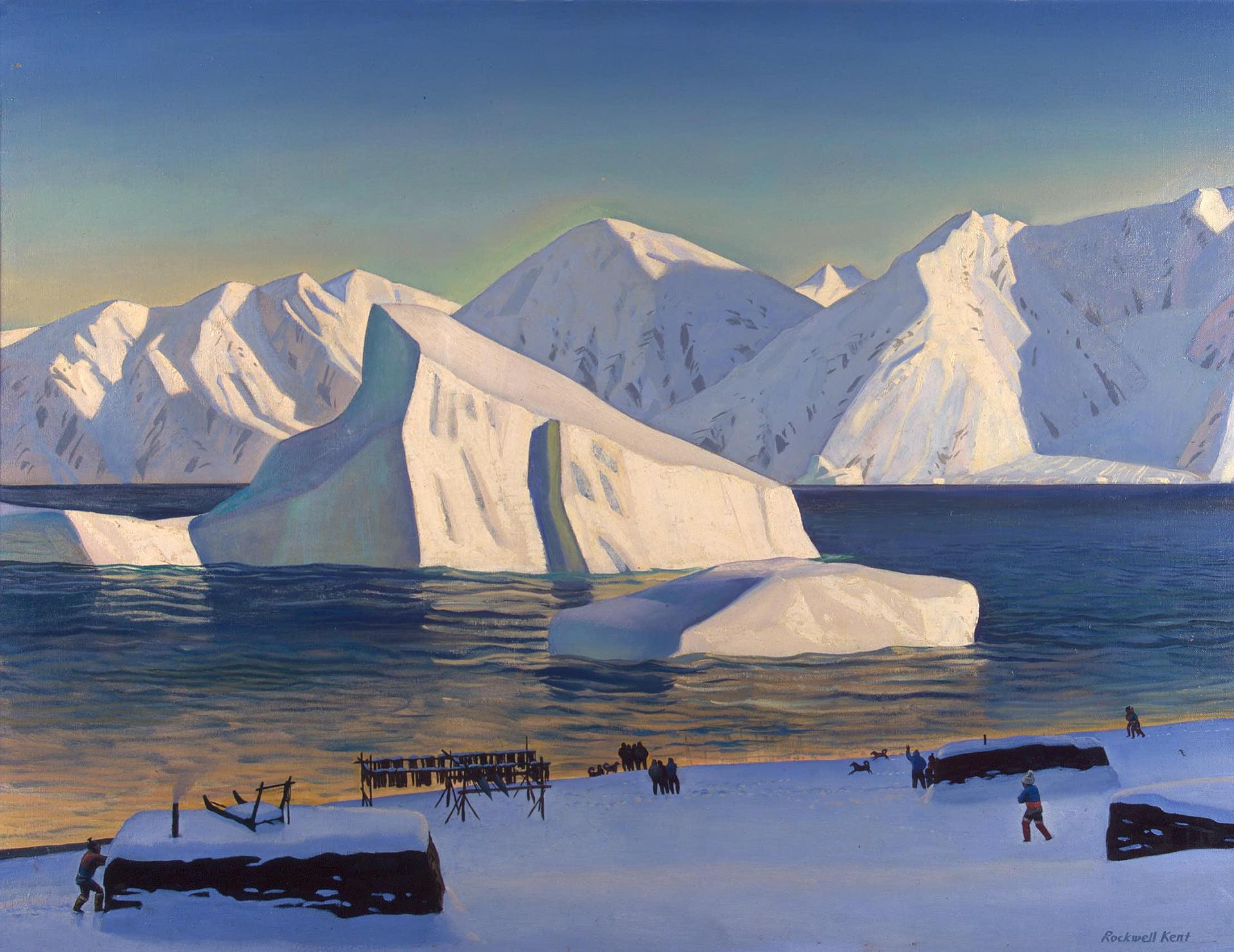The image depicts a winter landscape, possibly located in the Arctic or Antarctica, characterized by a dramatic interplay of icy blues and muted golds. The backdrop is a sky that transitions from dark blue at the top to a light blue-green and then to a golden hue near the horizon, suggesting a sunset. Dominating the background are large, towering snow-covered mountains. These mountains or ice caps do not appear to be in water, resembling majestic frozen hills with dark rocky bases peeking through the snow.

In the middle ground of the composition, a prominent glacier stands tall in the water, nearly matching the size of the distant mountains due to its closer perspective. To the right of this large glacier is a smaller chunk of ice, emphasizing the rough and jagged beauty of the frozen landscape.

The foreground features a snow-covered shoreline dotted with rectangular, almost hut-like structures that appear to be partially submerged in ice. These structures may serve as homes or shelters for the inhabitants. Small groups of people can be seen walking on the shoreline, some engaged in work near the huts, others closer to the water. There are even a couple of tiny dogs running along the shore, adding a touch of life to the serene and cold environment. Among the huts, one stands out with what seems to be a chair on its roof and a little smokestack, suggesting domestic activity inside. The still, reflective water near the shore captures the rich colors of the setting sun and the glacial reflections, enhancing the impression of an icy, yet inhabited, wilderness at the edge of the world.